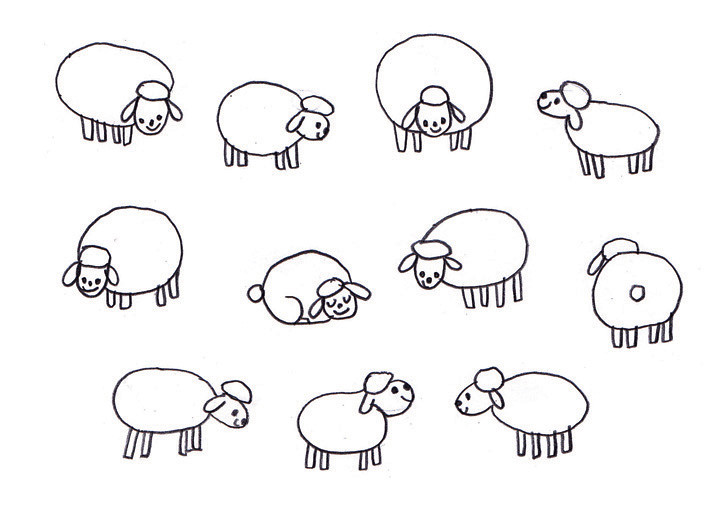The image shows a series of 11 simple, cartoonish doodle-style drawings of sheep, arranged in a landscape orientation without any background. The sheep are organized into three rows: four in each of the top two rows, and three in the bottom row. They are drawn in black ink, featuring oval or circular bodies, circular heads, and floppy oval ears. Each sheep has four rectangular, stick-like legs, a small circle of head fur, and dot eyes, button noses, with curved lines forming smiles. Most sheep are shown in profile, but some variations include one sheep lying down with closed, U-shaped eyes, another facing away with a visible round tail, and others facing different directions, enhancing the whimsical and amateurish feel, akin to a child's drawing or AI-generated art.